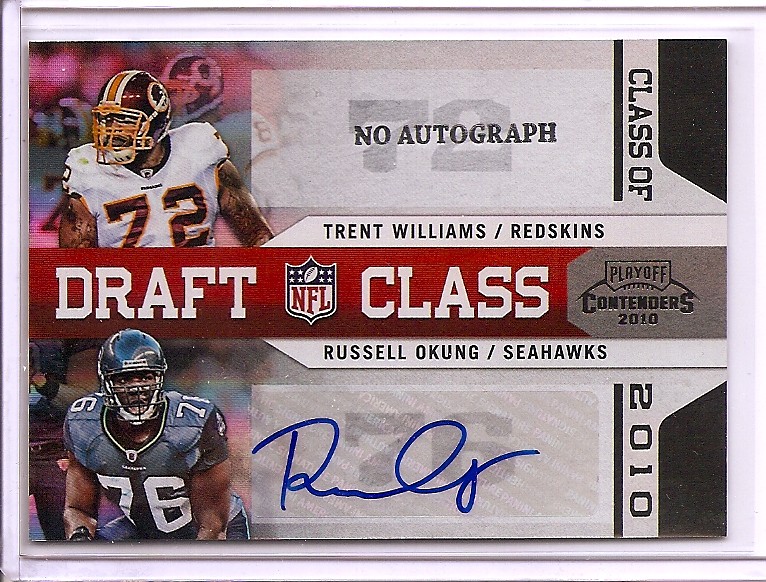The image showcases a framed football poster entitled "Draft Class Playoff Contenders 2010" against a white background. The poster features two football players, Trent Williams from the Washington Redskins at the top and Russell Okung from the Seattle Seahawks at the bottom. The left side of each player's section displays their color photographs—Williams in a white jersey and red helmet looking to the left, and Okung in a blue jersey and helmet looking slightly to the right.

A prominent red stripe bisects the poster vertically down the center, with the words "Draft Class" in white letters flanking the NFL shield logo, which has a white football at the top and four stars on either side. Below the NFL shield, "2010" is written in gray letters.

Above Williams' photo, "Trent Williams / Redskins" is written in black letters on a white background, with the number 72 grayed out behind the text. Notably, there is an empty space where his autograph should be, labeled "no autograph." Similarly, beneath Okung's photograph, his name "Russell Okung / Seahawks" appears above his signature in black letters, with the number 76 subtly visible in the background. Vertically along the right edge of the poster, the words "Class of 2010" are printed.